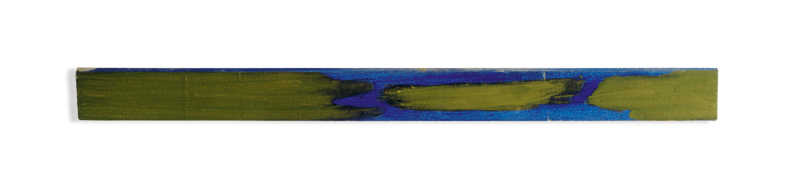The image is a horizontally oriented, narrow, and long rectangle dominated by varying shades of green, ranging from light to darker tones. The background contains a smudged green color with a few hints of darker green patches. Occupying the center of the canvas is an abstract shape that resembles a flipped letter "D," painted in different shades of blue; parts of this shape are lighter blue while others are darker. The blue shape has an uneven, cut-off edge on the left side. Accentuating the image are lines of blue paint: a longer line runs along the upper two-thirds of the canvas, while a shorter blue line is situated towards the very bottom. An additional dark blue horizontal band is visible further to the right, adding more depth to the composition. The image also features a white background towards the left, which transitions into the green color, contributing to the border-like appearance of the painting.